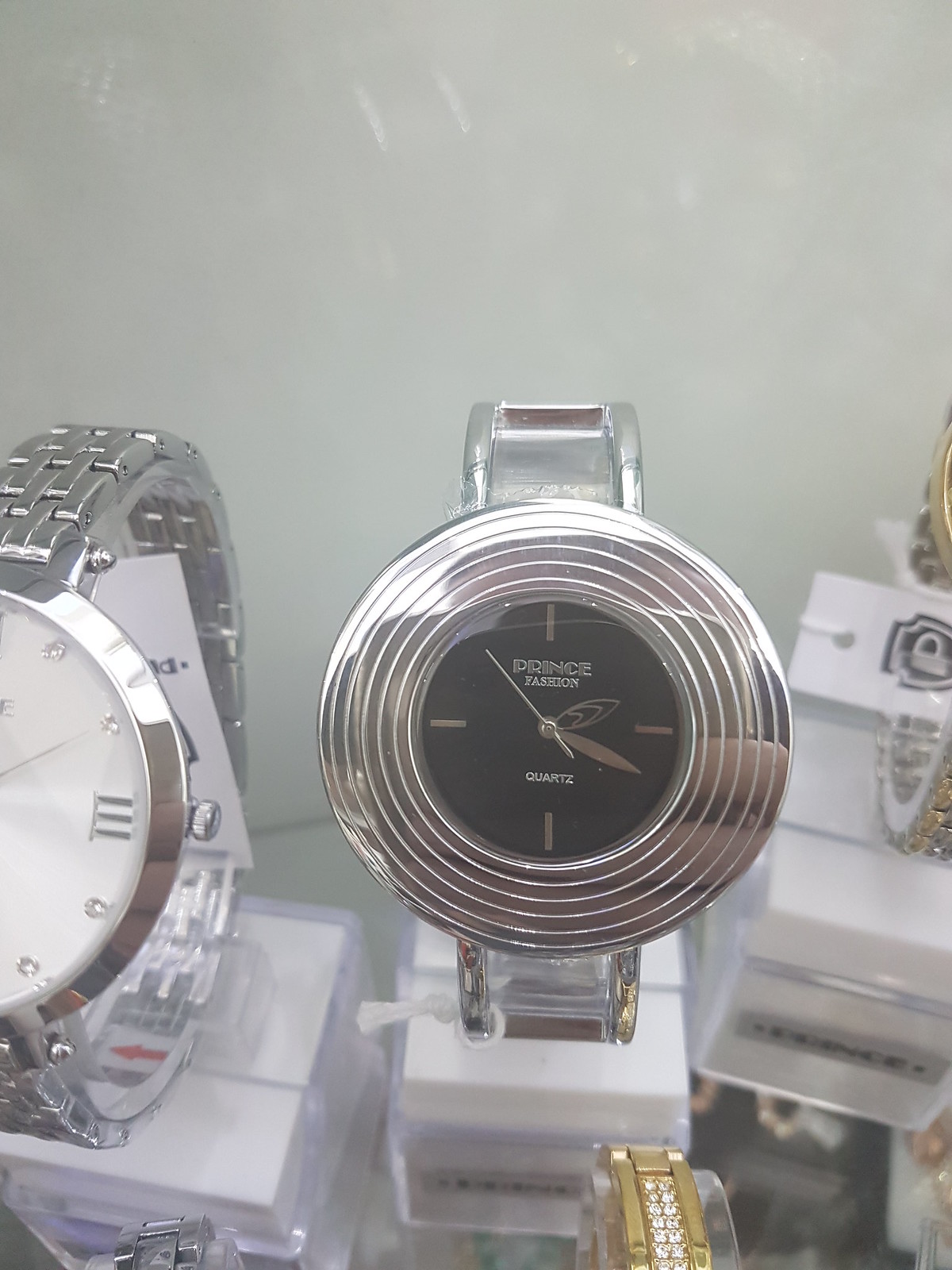In the image, there are five watches on display, each nestled upon white plastic stands within a glass display case, presumably in a watch store. The central focus is a distinctive silver metal watch with a black face. This watch features a circular face with unique rippling patterns extending outward from the center. The watch face is detailed with four gray and gold lines pointing to the cardinal directions, and the words "Prince Fashion" are prominently inscribed, followed by "Quartz" below. Additionally, a long, leg-like hand points towards the top left of the watch face. To the left of this central watch is another silver watch with a white face and a stretchable metal wristband. On the right side of the central watch, another silver watch can be observed. Partially visible below the center stand, there is a gold and diamond-banded watch, adding a touch of luxury to the display. The background of the display case is stark white, highlighting the elegance and diversity of the watches.